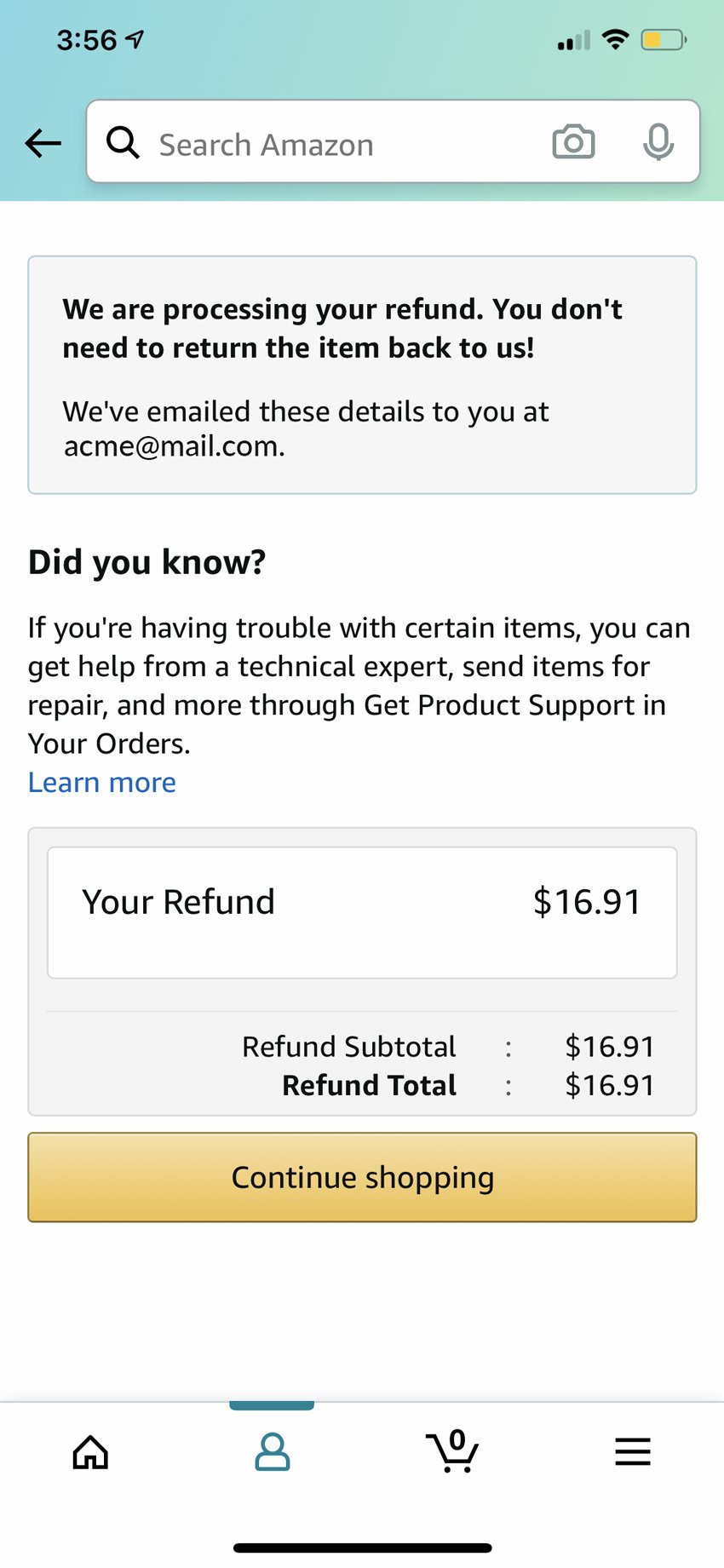The screenshot shows an Amazon app interface on a smartphone, indicated by the time "3:56" at the top left and the battery icon at the top right, which is slightly less than half-full and yellow. At the top of the screen, within the Amazon app, there is a search bar labeled "Search Amazon," which is currently empty.

Below the search bar, there is a gray notification box with a message in black text that reads: "We are processing your refund. You don't need to return the item back to us. We've emailed these details to you at acme@mail.com." Additionally, it offers assistance with problematic items, advising users that they can get help from a technical expert, send items for repair, and more through the "Get Product Support" option in their orders. The phrase "Learn More" appears in blue, clickable text, inviting users to gain more information.

Further down, the screen details the refund process with the text "Your Refund: $16.91," and below it, both the "Refund Subtotal" and "Refund Total" are listed as "$16.91." At the bottom of the notification, a yellow button with black text prompts the user to "Continue Shopping."